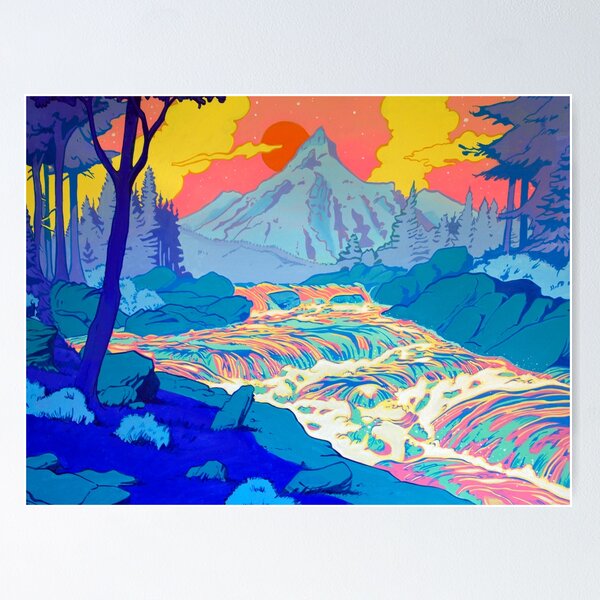This is a colorful and detailed painting of an outdoor scene, evocative of an artist's rendering. The sky in the background exhibits a vibrant blend of yellow, pink, and slight hues of blue, with an orange sun that contributes to the overall warm tone. The distant mountains are painted in pale blue with darker blue accents, providing a serene backdrop. Moving forward to the lower right portion of the image, there is a groundscape with gray stones and boulders, and notably, a tall tree without visible leaves, bifurcating into two separate branches.

Centrally, a powerful river demands attention as it cascades, forming a small waterfall in its course. The river's water is an eclectic mix of colors, including orange, tan, pink, white, blue, and purple, creating a dynamic and mesmerizing effect. Despite the absence of any signatures or text, the painting stands out with its use of pastels and vivid hues, highlighting blue trees and grass, providing contrast against the rocky terrain. The overall impression is one of a whimsical and enchanting landscape, skillfully brought to life with a delicate balance of colors and elements.